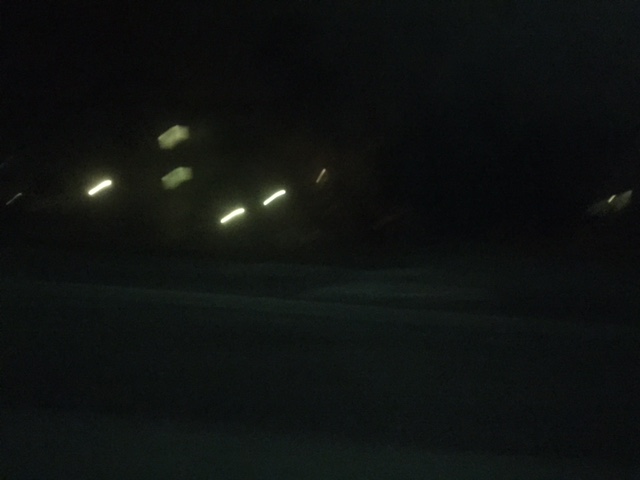The image, captured outdoors at night, is an almost completely black and blurry horizontal photo. The ground below is faintly visible and appears puffy, possibly covered with snow. Central to the image, there are streaks and bands of light extending horizontally across the center, with a section slightly off to the upper left where six light bars can be seen—three bright white and three faint and gray. These lights, possibly part of a distant hillside or building, are positioned at angles pointing upwards from the left to the center. To the right, there is a light splotch with a lighter dot, separate from the main light bands. The overall scene is enveloped in darkness, creating a mysterious and obscure view.